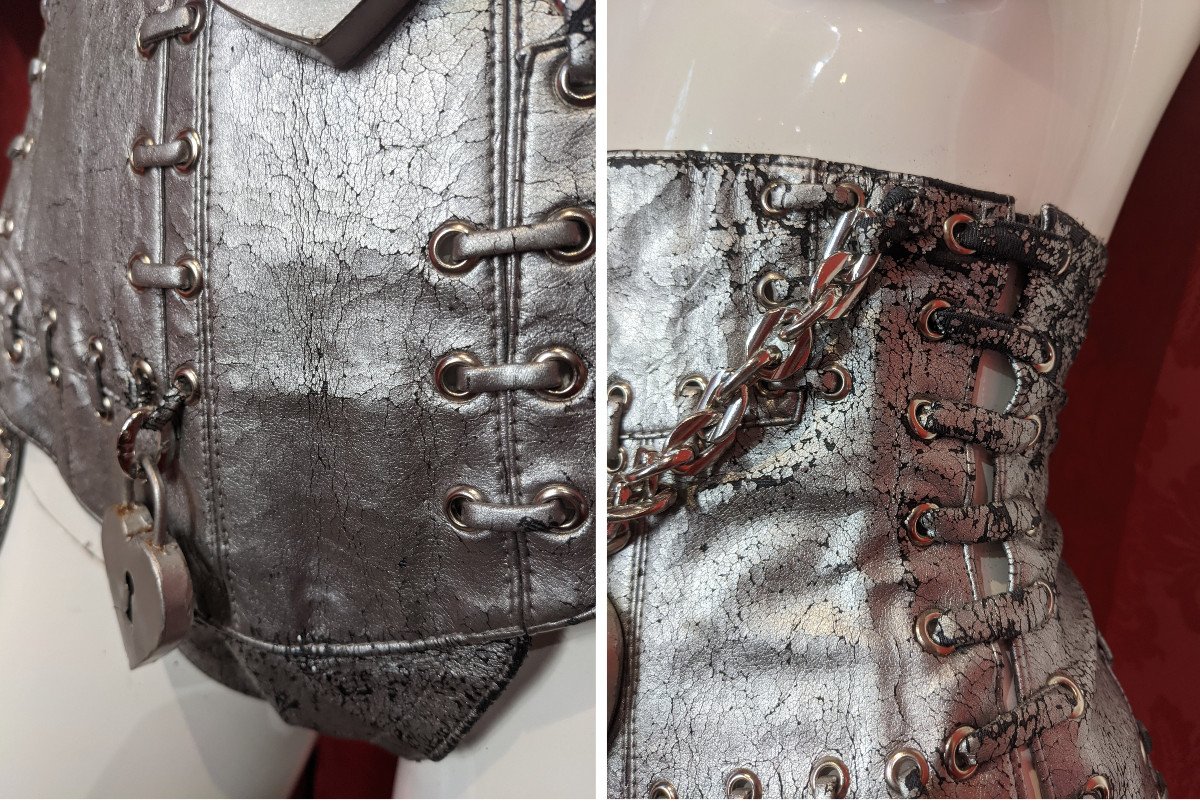The image depicts a metallic silver corset-like garment, potentially a chastity vest, showcased in a museum setting. The corset features multiple latches for fastening, without any buttons, and is equipped with a distinctive heart-shaped lock, which has an old-fashioned keyhole. This lock, possibly serving to secure the garment in place, adds an intriguing element to its design. The corset appears aged and cracked, extending to include a crotch area. Numerous holes with lacing are threaded through them, complemented by silver rings throughout the garment. A silver chain dangles from it, enhancing its complex and intriguing appearance. The background includes red curtains and white walls, further emphasizing that this item is on display in an exhibit.